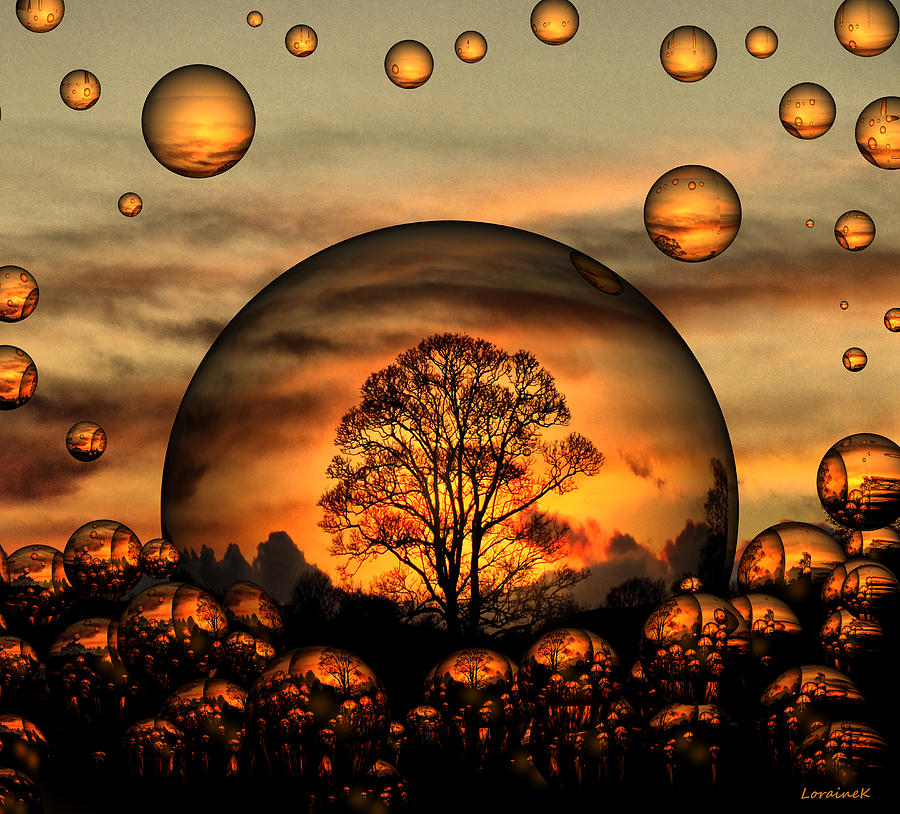This image is an artistic rendering signed by Lorraine K. in the bottom right corner. The composition features a surreal, bubble-filled landscape set against a vivid backdrop resembling a cloudy sunrise or sunset. In the center of the image is a large, prominent bubble containing a dark, almost black silhouette of a bare tree, with jagged rock formations reminiscent of a canyon below, and a dreamy sky with hints of blue and varying cloud formations in the background. Surrounding this central bubble are numerous smaller bubbles scattered across the scene, each reflecting segments of a nature landscape that echo the central image but vary slightly in detail. The predominant colors are shades of amber, dark browns, and blacks, with warm reds, yellows, and touches of blue adding depth and contrast. The lower portion of the image is densely populated with these bubbles, overlapping and differing in size, creating a fantastical mosaic that blends elements of nature and abstract art.